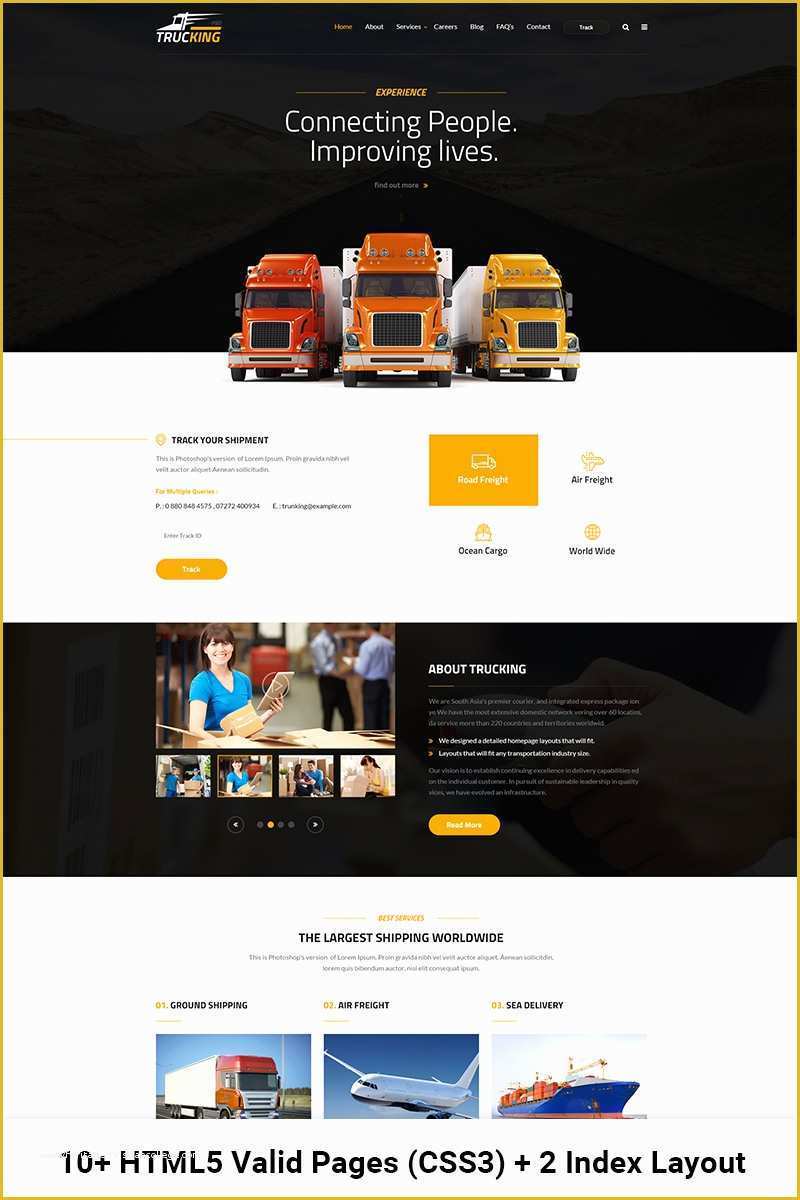The image showcases the front page of a professional trucking company's website named "Trucking King." At the top left corner, "Trucking" is displayed in white, and "King" in gold, with a silhouette of a truck cab above it. Adjacent to this logo are navigation buttons labeled Home, About, Blog, and other sections, all rendered in small white text. Centered prominently on the page is the word "Experience" in gold, followed by the tagline "Connecting People, Improving Lives" in larger font.

Below this tagline, three tractor-trailers are parked side by side: a red one on the left, an orange one in the center, and a gold one on the right. Each trailer is white and rectangular. Underneath this, there is a section titled "Track Your Shipment," accompanied by small black text and four buttons, each with distinct yet diminutive logos.

Further down is an "About Trucking" section, featuring white text on a black background. Beside the text is a collage of four photographs, with the most prominent being a Caucasian woman smiling at the camera. She has brown hair, wears a blue blouse, and holds a tablet in one hand and a box in the other.

Continuing below, there's a section titled "The Largest Shipping Worldwide" with three separate images: a red truck with a white cargo on the left, an airplane in the center, and a large blue cargo vessel on the right. At the bottom of the page, a text block mentions "10+ HTML5 valid pages" and "CSS3 + 2 index layouts," in black text on a white background.